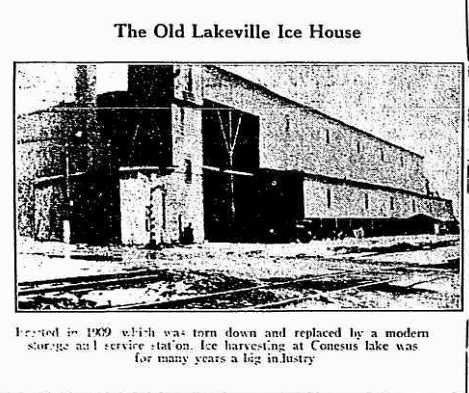The photograph is a black-and-white, grainy image likely scanned from an old newspaper or book, depicting "The Old Lakeville Icehouse," as indicated by the black text at the top. The picture shows a large, industrial building that is approximately three stories tall, dominating most of the frame. On the right side of the building, which has two distinct layers, there are two sets of windows—one at the top and one at the bottom, totaling about ten windows. The building features a large open bay, presumably for deliveries and exports. In the foreground, two sets of railroad tracks and a road intersect the tracks moving diagonally from the bottom left to the bottom right of the image. Below the photograph, a partially legible caption reads, "Erected in 1909, which was torn down and replaced by a modern storage and service station. Ice harvesting at Consenus Lake was for many years a big industry," although parts of the text are faded and unreadable. The image, overall, captures a piece of industrial history with visibly aged and distressed quality.